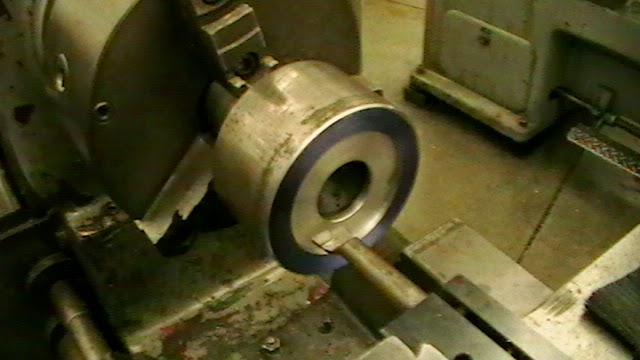The image captures a close-up of an industrial workshop scene, focusing on a complex piece of machinery that is primarily cylindrical in shape. At the center of the machinery is a prominent circular part with a hole, potentially designed to hold or process materials. Surrounding this central feature are blades or component parts indicative of a mechanical function. Attached to this is a larger cylindrical metallic piece.

The lighting in the image casts an almost letterless, olive-yellow tint over the entire scene, which complements the industrial, metallic ambiance. Located in the upper and lower right sections of the frame are additional mechanical components, including a thicker pole and a foot-operated mechanism, likely for controlling the machinery. Bolts and nuts are visible in the lower left, hinting at the machine's assembly or maintenance features, while the background reveals another large, nondescript metal machine, adding layers to the industrial setting. The floor is tiled, and the overall color palette is dominated by shades of yellow and olive, reinforcing the utilitarian atmosphere of the workshop.